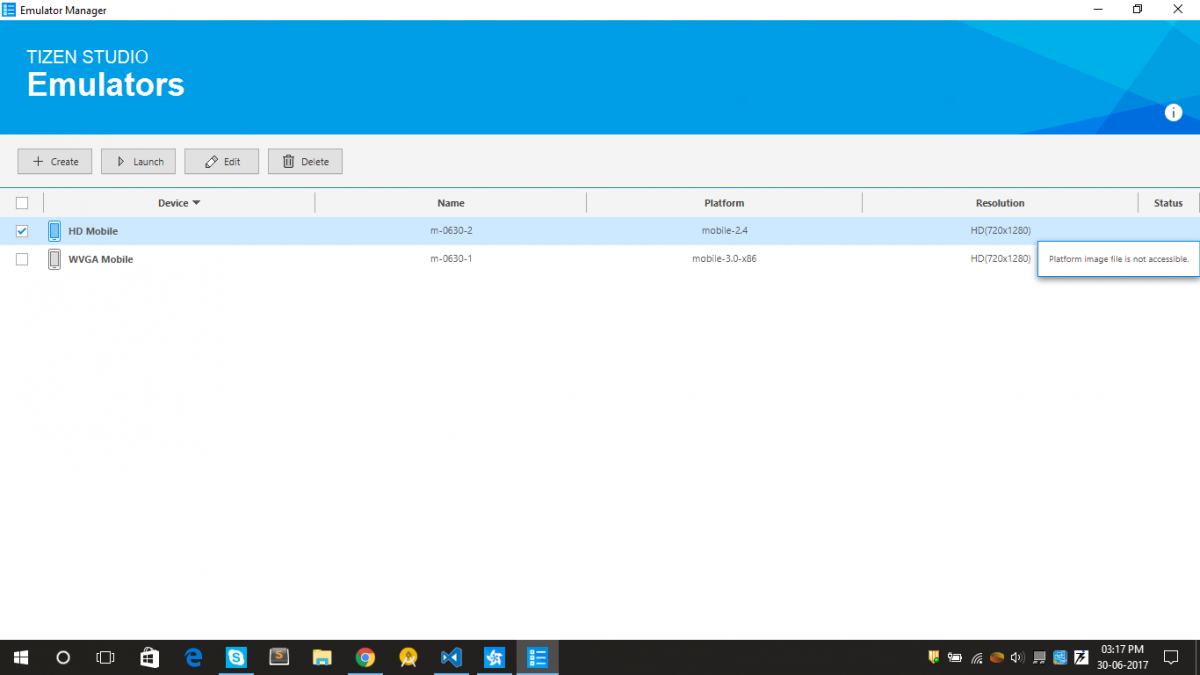The image is a detailed screenshot of a computer screen displaying the Emulator Manager program within Tizen Studio Emulators. The interface features a primarily white background with a blue header. Within the program, several buttons are prominently displayed, including 'Create,' 'Launch,' 'Edit,' and 'Delete.' Listed under the available devices section are two entries: 'HDMobile' with a blue checkmark indicating its status, and 'WVDAMobile.' The latter includes additional details such as the name, platform, and resolution, along with a note indicating that the platform image file is not accessible.

At the bottom of the screen, a black taskbar is visible, featuring various icons for launching different desktop programs. This taskbar also displays essential system notifications including battery percentage, Wi-Fi connectivity, volume control, and the current time and date. A small messaging icon is also present. The overall layout is clean, delineated clearly by the program's blue and white color scheme, offering a user-friendly interface for managing emulator settings.